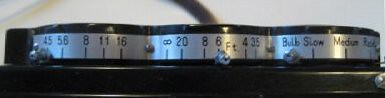This photograph captures a detailed, almost panoramic view of a sophisticated camera lens. The image focuses on the side profile of the lens, revealing a meticulously designed cylindrical structure marked by a silver ribbon running along its circumference in a semicircular pattern. This reflective silver band is etched with measurement indicators, including 45, 58, 8, 11, 16, followed by 28, 6, 4, and 3.5, which appear to be distance scales measured in feet. Additionally, one segment is labeled with terms such as 'bulb,' 'slow,' and 'medium,' though the final part of this section remains partially illegible.

The predominantly black lens exterior is made from a metal material that gives off a reflective sheen, and its sleek construction is accentuated by a series of visible screws that secure its components together. The bottom portion, also made of metal, integrates seamlessly into the overall design, emphasizing the precision engineering typical of high-quality photographic equipment. This lens, likely an essential tool for professional photographers, exudes a sense of durability and meticulous craftsmanship, capturing both form and function in this artfully framed shot.